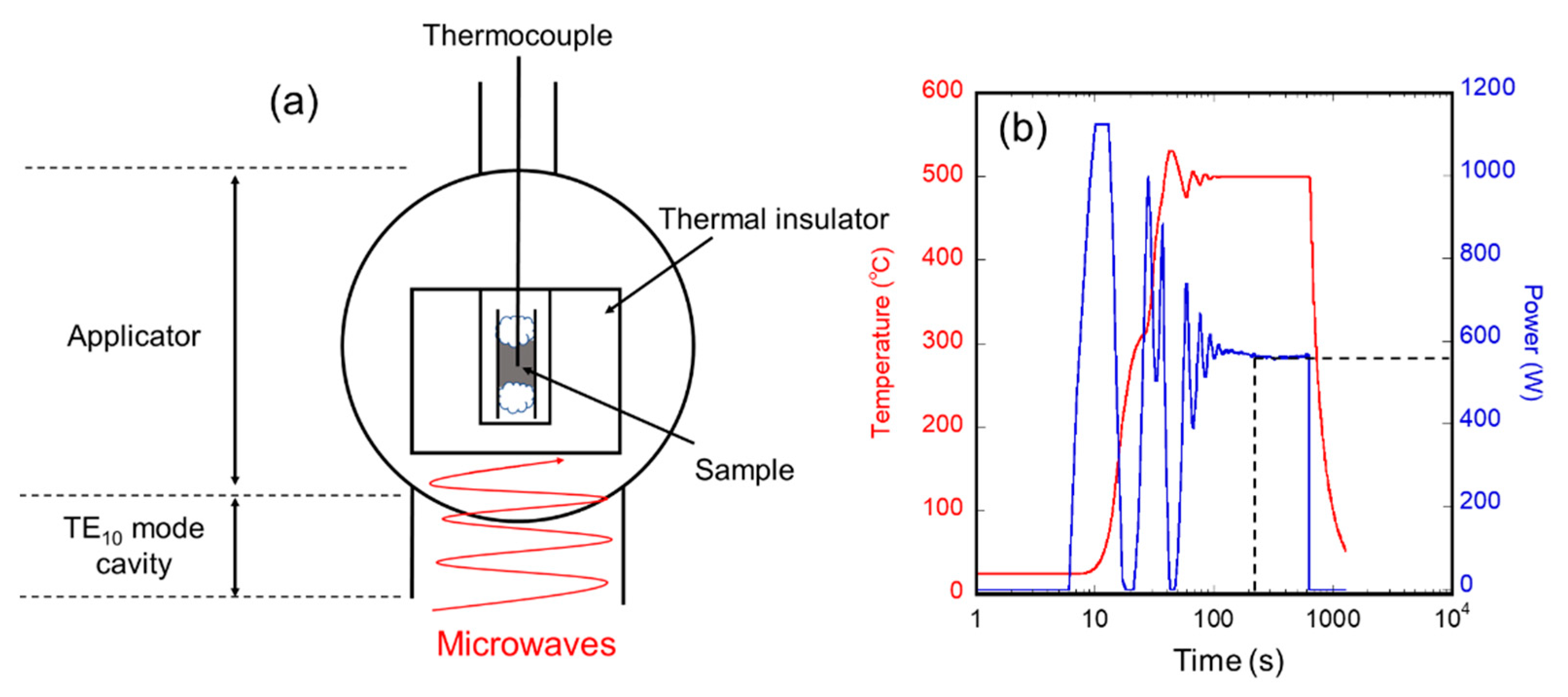The image is a detailed diagram on a white background with no border, utilizing predominantly black coloring with accents of red and blue. On the left side, the diagram focuses on microwaves, featuring a black-outlined circle that encloses a vertical rectangle labeled as a thermocouple. This rectangle contains two diagrams with lines originating from a cloud-like top and bottom section, shaded gray in the center. Surrounding this figure is another rectangular section labeled as a thermal insulator. Below this setup, a red wavy line is identified as microwaves, which are labeled in red. Adjacent to it, the term “applicator” and the notation “TE10 mode cavity” is indicated.

To the right of this assembly sits a vertical graph characterized by jagged lines in red and blue. The vertical axis on the left side represents temperature in degrees Celsius, with increments from 0 to 600, plotted in red. The right vertical axis represents power measured in wattage, with increments from 0 to 1200, plotted in blue. The horizontal axis at the bottom spans from 1 to 1000 in logarithmic scale, marked 1, 10, 100, and 1000, denoting time.

This diagram integrates comprehensive elements of microwave interaction, thermal insulation, and energy metrics graphically represented with a correlation between temperature and power over time.